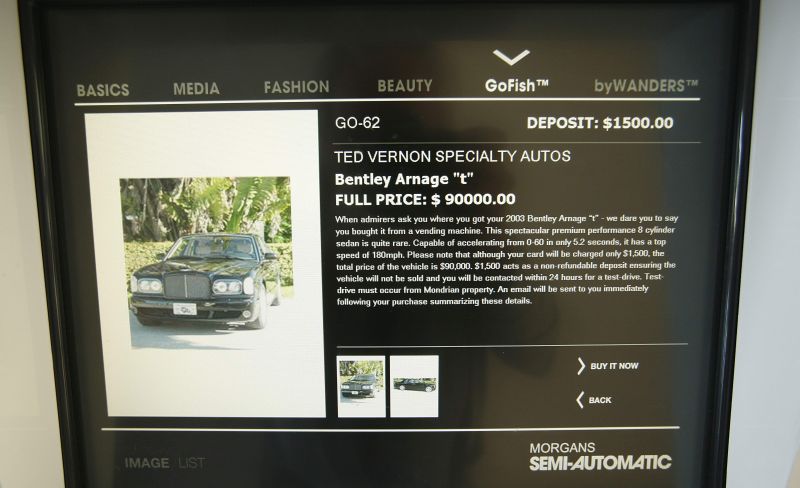The image depicts a screenshot of a webpage featuring a black Bentley Arnage T. The webpage is populated with various tabs including "Basics," "Media," "Fashion," "Beauty," "Go Fish," and "Buy Wonders," all set against a grey or white background. Prominently displayed in the center is a color photograph of the Bentley Arnage T, a premium 8-cylinder sedan capable of accelerating from 0 to 60 mph in just 5.2 seconds and reaching a top speed of 180 mph. The text highlights its rarity and luxury. The listing specifies a "Full Price: $90,000" and includes markings such as "Go $62," "Deposit $1,500," and the dealership name "Ted Vernon Specialty Autos." The interface features buttons for "Buy It Now" and a "Back Button," indicating it's an interactive purchase page. The colors primarily present are black, white, grey, and green.